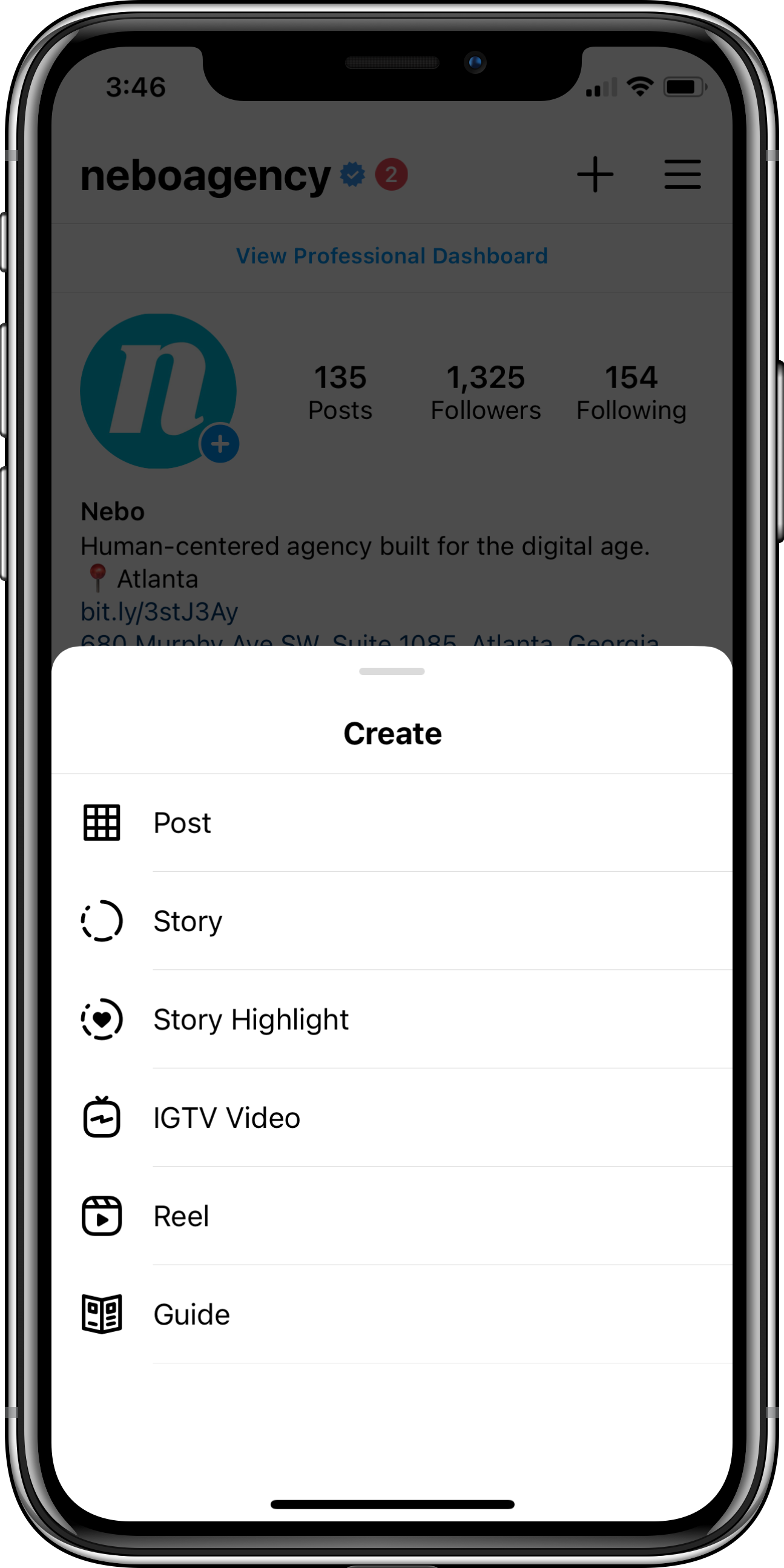The image captures a screenshot taken from the front of someone's cell phone. The main focus is a pop-up interface at the bottom of the screen featuring a "Create" area, which is displayed in white. Running down the left side of this rectangular area are six icons with corresponding labels. From top to bottom, the icons and labels are as follows:

1. A checkerboard icon labeled "Post".
2. A dotted circle icon labeled "Story".
3. A heart icon with a dotted circle line around it labeled "Story Highlight".
4. A television set icon labeled "IGTV Video".
5. A movie clapperboard icon labeled "Reel".
6. A booklet icon labeled "Guide".

In the background, partially visible, is a screen showing text and information presumably from a social media profile. It displays:

- The name "Nebo Agency" accompanied by an icon of a lowercase white 'n' within a blue circle.
- Metrics indicating "135 posts", "1,325 followers", and "154 following".

These elements provide an impression of a user interacting with a social media app, specifically in the section where content creation options are available.